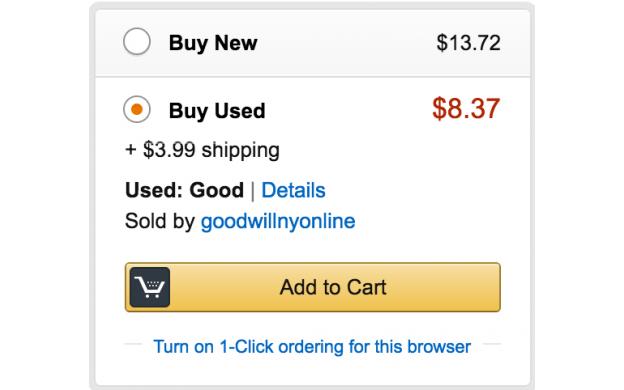The image depicts a small pop-up window typically seen on an e-commerce website. The background is gray over a white field. At the top of the window, there is an option labeled "Buy New" with a selection circle next to it. The "Buy New" option is priced at $13.72 and is underlined by a thin gray line.

Below this, there is another option labeled "Buy Used," which is currently selected, indicated by a yellow dot inside the selection circle. The "Buy Used" option is priced at $8.37, with an additional $3.99 for shipping. This item is described as "Used; Good" in red text. 

Underneath the price and condition, there is a "Details" link in blue text, followed by the seller information, "Sold by Goodwill NY Online," also in blue text. Both the "Details" link and the seller information are clickable.

At the bottom of the pop-up window, there is a bright yellow "Add to Cart" button, featuring a shopping cart icon within a black square to its left. Below this button, in blue text, is a prompt that reads, "Turn on 1-Click ordering for this browser," which is also a clickable link.

The entire content is set against a simple white background with no indication of the specific website.